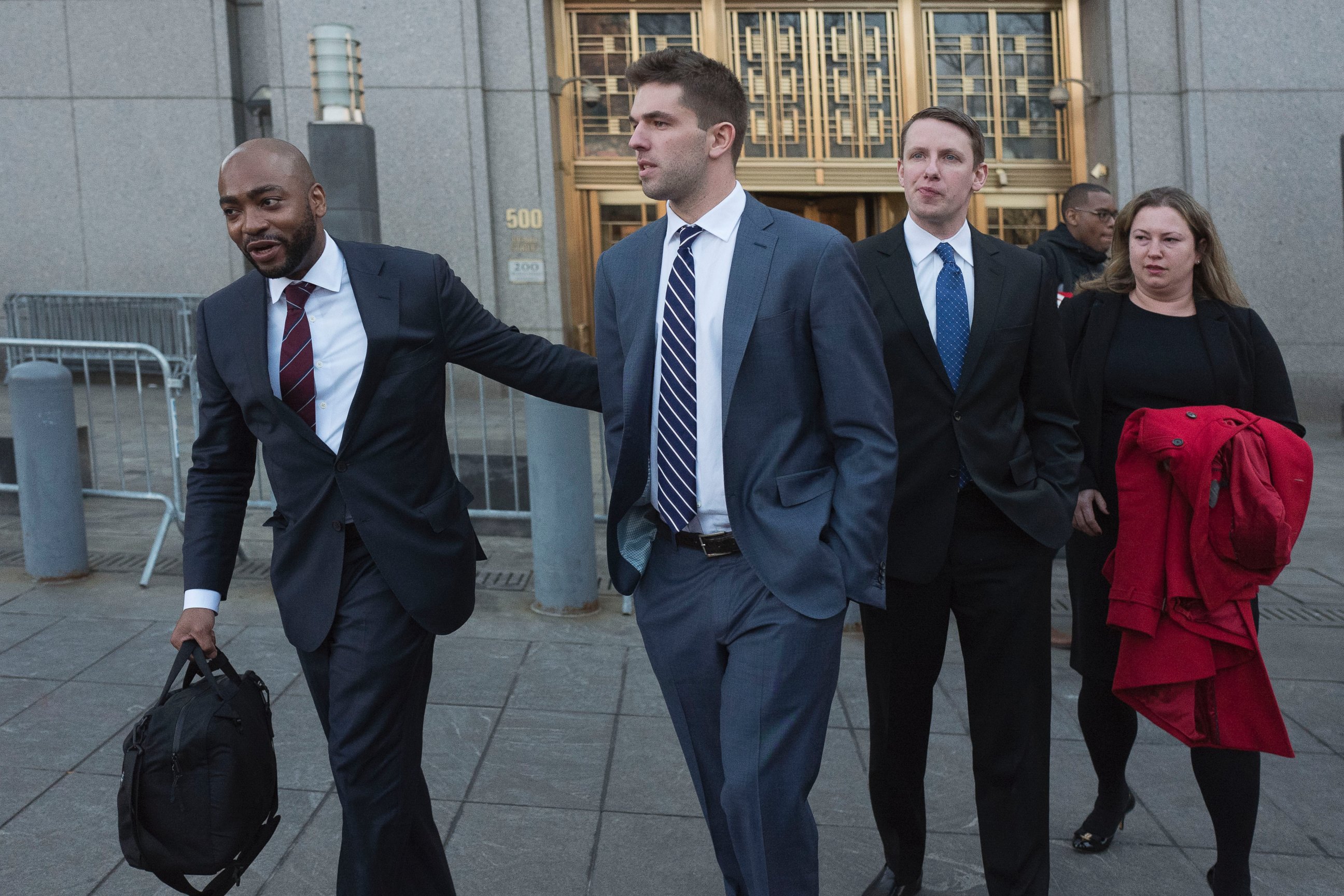In this outdoor scene, a diverse group of individuals appears to be exiting a formal building resembling a courthouse or office, located at an address prominently marked "500" in gold font above a large golden glass doorway. The scene is dimly lit despite being daytime, with concrete surfaces and metal barriers structuring the pathway. The group includes a white man in his late 20s to mid-30s wearing a gray suit, white shirt, and a dark blue and white striped tie; another white man in a black suit, white shirt, and blue tie; and an African-American man, perhaps in his 30s, with a shaved head, beard, black suit, white shirt, and red tie, who is carrying a black briefcase in his right hand and has his arm behind the man in the gray suit. Additionally, there is a woman, dressed in black, possibly in her late 30s or early 40s, holding a bold red coat. In the distant background, another African-American man is seen, though it is unclear if he is part of the group. This scene, with its formal attire and setting, gives the impression of a legal team escorting a defendant out of a courthouse.